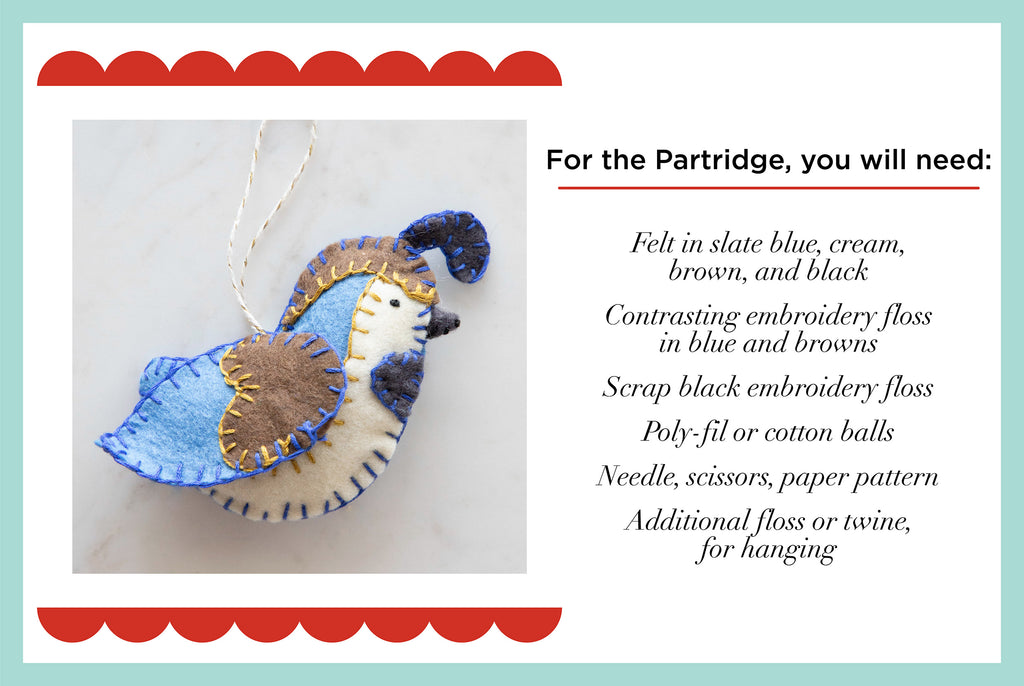This detailed infographic, resembling a PowerPoint slide, features a DIY guide for creating a charming handmade partridge Christmas tree ornament. The image is set against a white background framed by a light blue rectangular border. The central focus on the left is a meticulously crafted felt partridge, stitched together with visible seams, displayed on a gray backdrop. This bird, facing right, showcases a mix of blue, brown, and white hues with distinct details: blue and brown wings, a white chest, a brown head crowned with a small black feather, a black beak, and a black accent on the chest. Red wavy semicircle designs embellish the top and bottom of its square photograph, adding a festive touch.

On the right side, the black text begins with a bold heading underlined in red, "For the partridge you will need," followed by a list of required materials in italicized black text. The listed materials include felt in slate blue, cream, brown, and black; contrasting embroidery floss in blue and browns; scrap black embroidery floss; polyfill or cotton balls; needles; scissors; a paper pattern; and additional floss or twine for hanging. This detailed list ensures that anyone can recreate this delightful ornament by following the comprehensive guide provided.